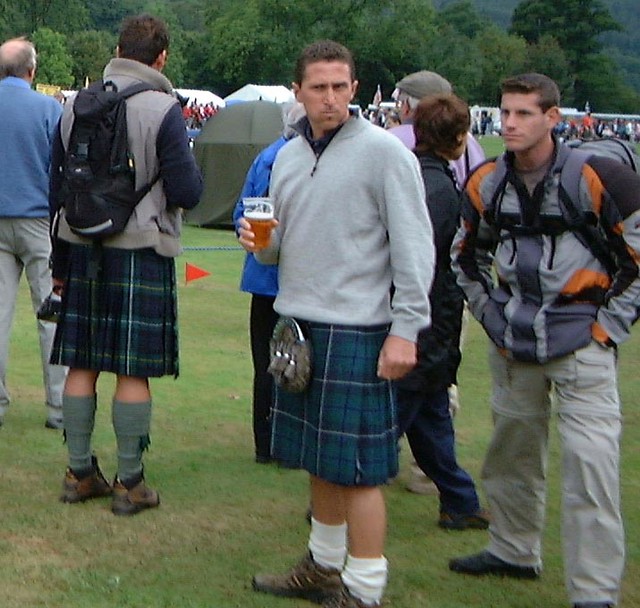This color photograph captures a vibrant scene at what appears to be a cultural fair or gathering in a park, with a lush green lawn and a backdrop of thick, dark-green trees. Several tents of varying colors—white, light blue, and dark green—pepper the background, along with a conspicuous red flag planted in the ground. The day is bright, allowing for clear visibility of the various attendees scattered across the field, some in traditional Scottish attire, others in casual or athleisure wear.

Front and center is a man in a blue tartan kilt, prominently featuring a silver sporran adorned with tassels. His outfit includes a gray zip-neck sweatshirt, white socks, and short hiking boots. He stands close to the camera, gripping a half-drunk pint of brown beer, his face contorted into a glower with furrowed eyebrows and pursed lips. To his left, another man also wearing a kilt, this one chiefly dark blue with white, green, and yellow stripes, faces away from the camera. This individual pairs his kilt with a long-sleeved dark blue t-shirt, green socks, and brown shoes with black soles.

In addition to these central figures, the scene includes a partly bald man in a blue sweatshirt and gray pants, a person in a white or gray vest, and multiple other attendees in jackets, backpacks, and pants of various colors. The crowd seems engaged in different activities, with some focused on a bagpipe or drumming performance happening some distance away. The photograph exudes the atmosphere of camaraderie and festivity, accentuated by the blend of traditional and modern attire set against a picturesque outdoor backdrop.